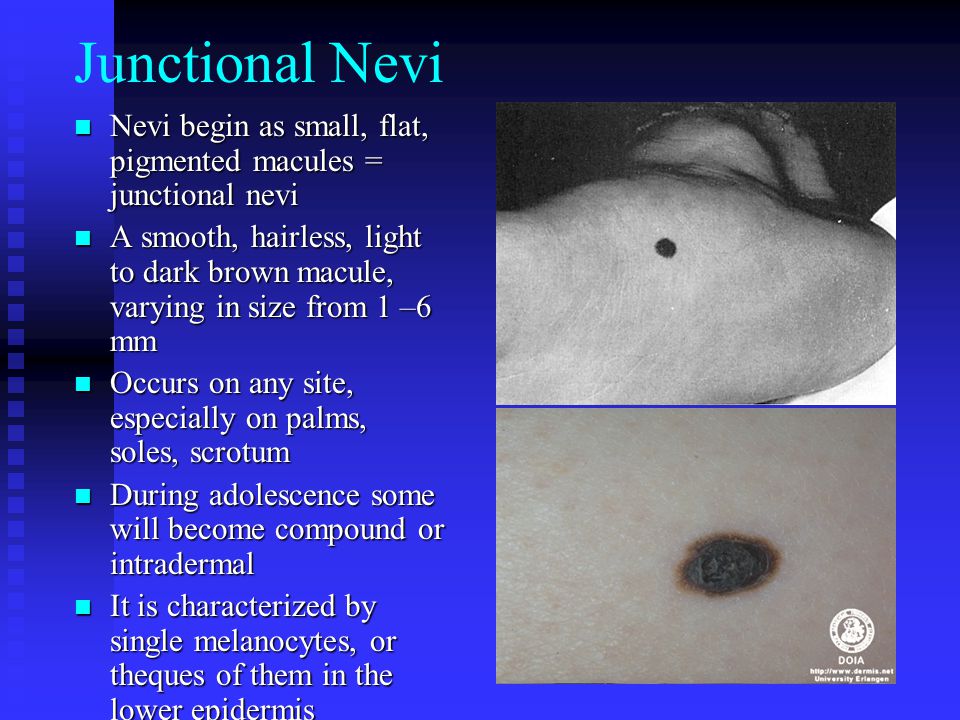This detailed image appears to be from a medical presentation or informational infographic, likely depicting junctional nevi, a type of mole or skin lesion. The visual layout includes two main close-up images positioned on the right side: a larger black and white photograph of what seems to be a foot with a small mole, and a magnified view of this mole below it. The images show varying shades of gray, black, white, as well as light and dark blue, and purple.

On the left side of the image, there is detailed text formatted with square bullet points, elaborating on junctional nevi. The topmost bullet points state that nevi begin as small, flat, pigmented macules, which are smooth, hairless, and light to dark brown, varying in size from 1 to 6 millimeters. Following this, the text explains their common occurrence on any body site, but especially on the palms, soles, and scrotum. The next points mention that during adolescence, some nevi may develop into compound or intradermal forms, and are characterized by single melanocytes or clusters of them in the lower epidermis.

The overall design and detailed medical content suggest this image could be part of a PowerPoint slide or educational pamphlet intended for medical use, possibly within a doctor's office or dermatological setting. The entire background is interspersed with colors including black, dark blue, and light blue, adding visual distinction to the educational material.